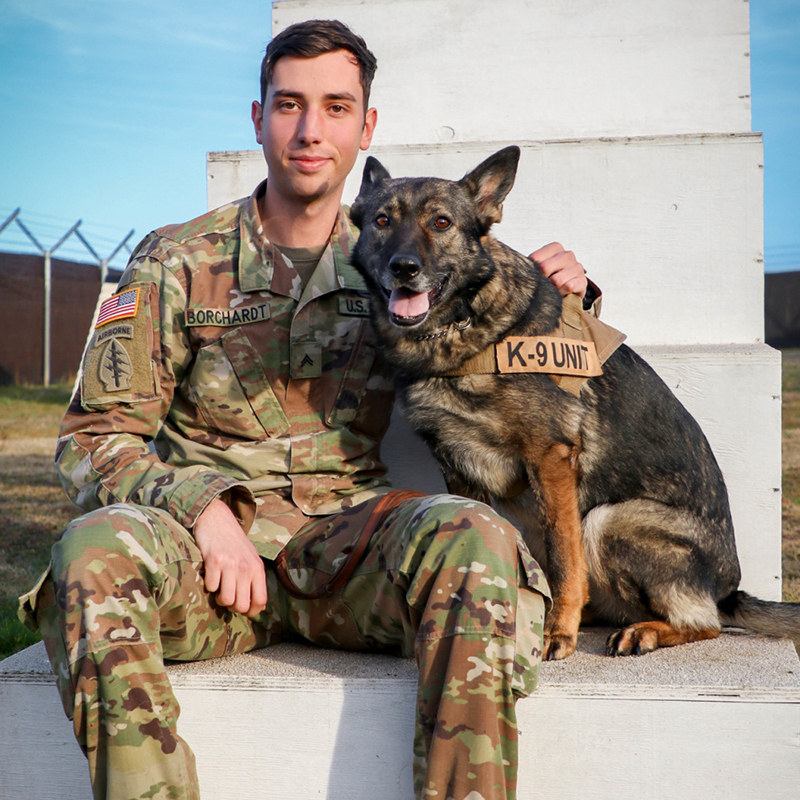This close-up photograph captures an army soldier seated on wooden steps alongside his canine unit. The soldier, identified by the name patch "Borchardt" on his fatigues, dons an army uniform complete with a USA flag patch and an airborne patch on his left forearm. He is a white man with short brown hair and a distinct birthmark on his chin. With a subtle smile, he gazes directly at the camera, exuding a sense of camaraderie with his canine companion.

The dog's breed appears to be a German Shepherd or Belgian Malinois mix, showcasing a coat that's black, tan, and whitish. Adorned in a tan vest labeled "K-9 Unit," the dog mirrors the soldier's steadiness, looking straight into the camera with its ears perked up and mouth open, as though panting. The leather leash, a key detail, drapes over the soldier's lap, while his right arm is casually placed on the dog's back.

In the background, a barbed wire-topped fence suggests an army base setting, reinforcing the disciplined yet close bond between the soldier and his loyal canine partner. The scene, infused with mutual respect and teamwork, offers a poignant glimpse into their dynamic duo.